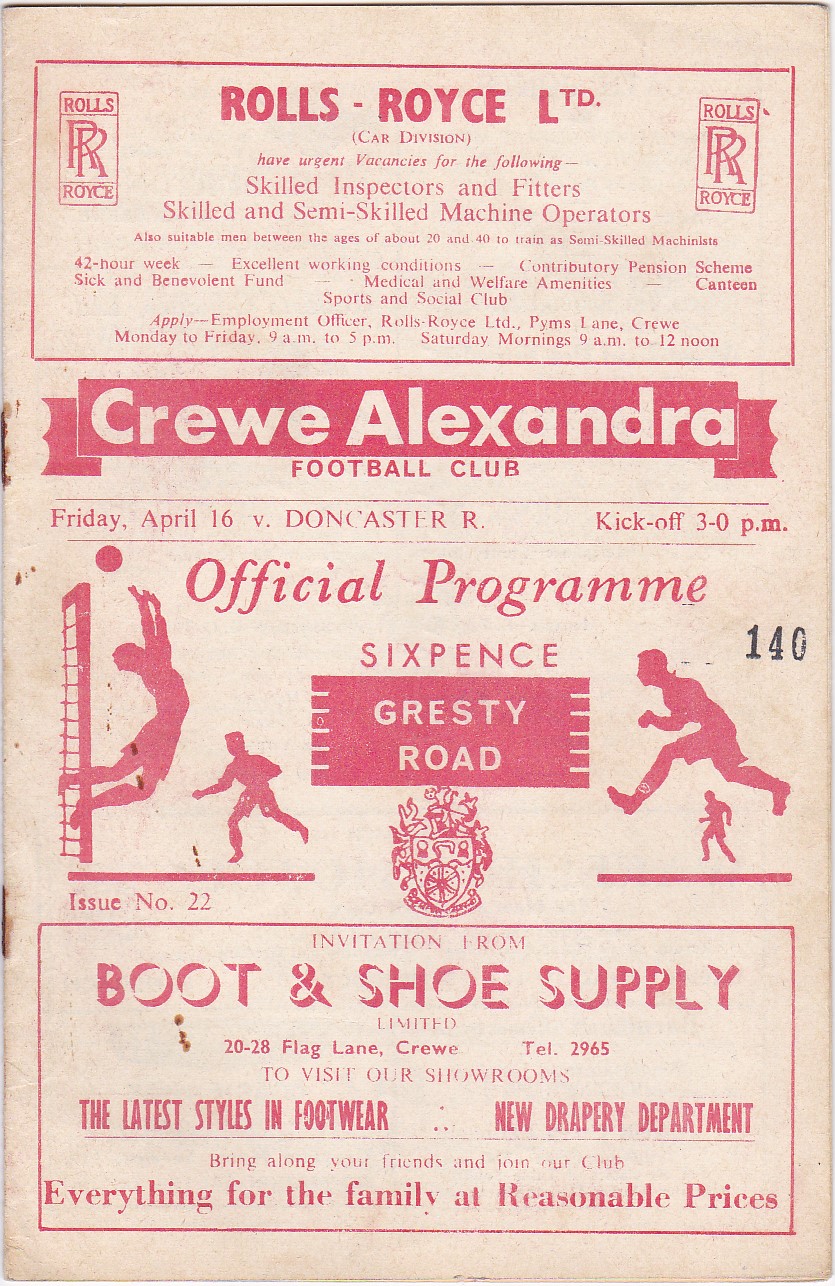The image appears to be an aged, off-white cover of an official event program or magazine, marked by multiple red text advertisements and announcements. At the top, a rectangular banner features an employment advertisement for Rolls Royce Limited's Car Division, seeking skilled inspectors, fitters, and semi-skilled machine operators. Detailed within are the job specifics, including a 42-hour work week, excellent working conditions, and various amenities, instructing applicants to visit their Pimms Lane Crew location from Monday to Friday, and Saturday mornings.

Central to the image is the main event highlight, showcasing "Crew Alexandra Football Club vs. Doncaster R." slated for Friday, April 16th, with a kick-off at 3 p.m. This section underscores the prominence of the football match in the program.

Towards the bottom, another ad from "Boot and Shoe Supply" promotes the latest styles in footwear, hinting at a new drapery department. The program notably includes issue number 22 in red text, adding a touch of period authenticity to the vintage document.